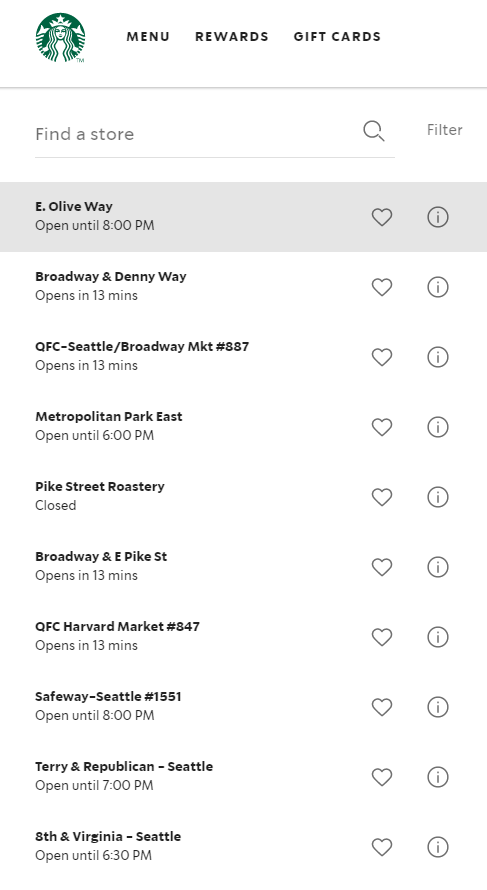A person is viewing their Starbucks app on a mobile device, searching for a nearby store to get a sweet treat. On the left side of the screen, the iconic Starbucks logo, featuring a white mermaid with long hair on a green background, is clearly visible. The app's menu displays several options in black text on a white background, including "Menu," "Rewards," and "Gift Cards." Below these options is the search functionality, complete with a magnifying glass icon and a "Filter" option.

The screen lists multiple nearby Starbucks locations, each accompanied by operational information and selection options:
- **East Olive Way:** Open until 8 p.m.
- **Broadway and Denny Way:** Opens in 13 minutes.
- **QFC Seattle Broadway Market (Store #887):** Opens in 13 minutes.
- **Metropolitan Park East:** Opens at 6 p.m.
- **Pike Street Roastery:** Closed.
- **Broadway East Pike Street:** Opens in 13 minutes.
- **QFC Harvard Market (Store #847):** Opens in 13 minutes.
- **Safeway Seattle (Store #1551):** Open until 8 p.m.
- **Terry and Republican Seattle:** Open until 7 p.m.
- **8th and Virginia Seattle:** Open until 6 p.m.

Each store listing features options to mark it as a favorite with a heart icon and to view more information with an eye icon inside a circle. The individual has highlighted the first option, East Olive Way, which is currently open until 8 p.m.